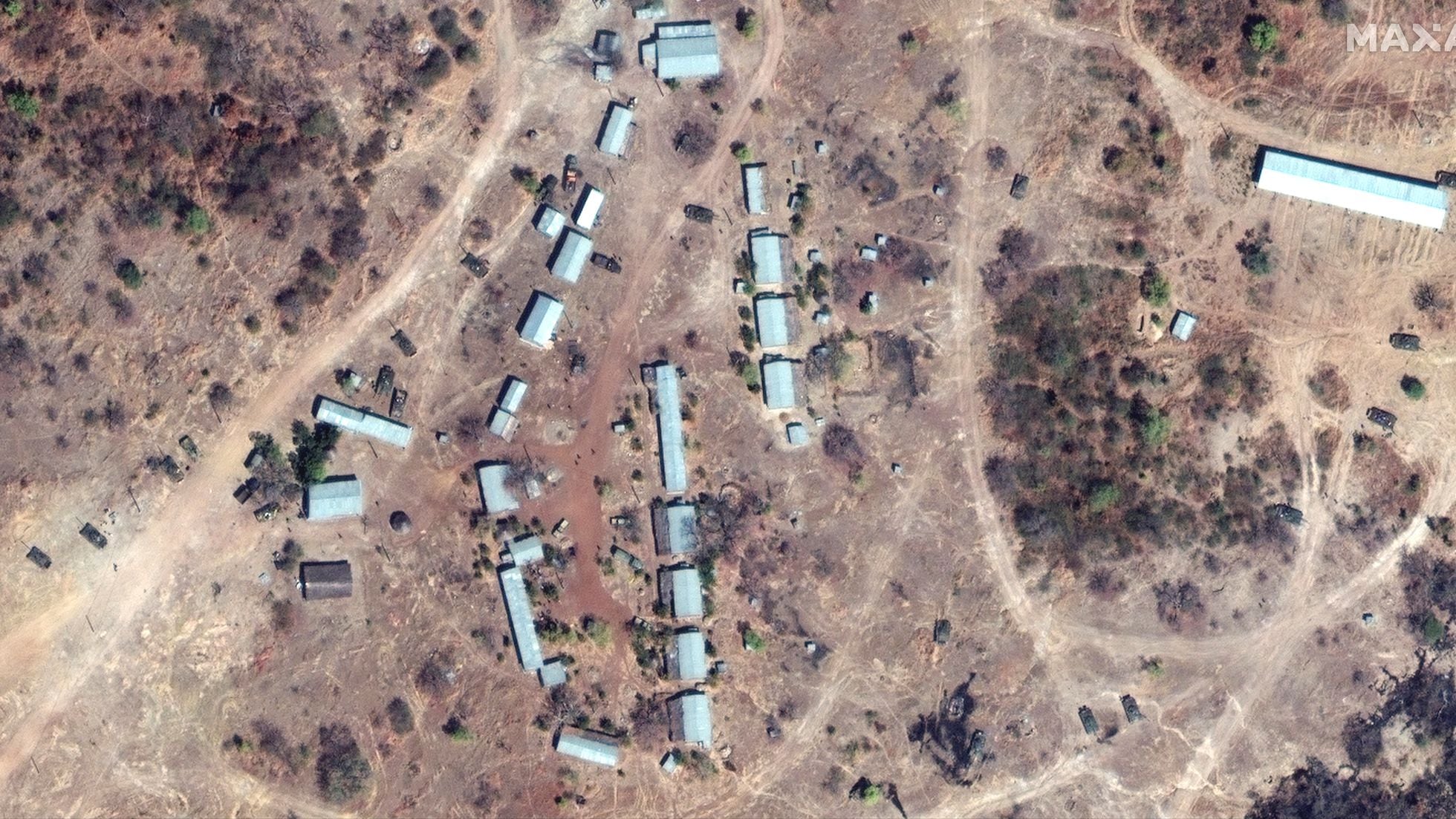The image displays an aerial photograph, possibly sourced from Google Maps, depicting a remote compound in a desert-like landscape with sparse vegetation. The terrain is predominantly dry and dusty, featuring a reddish tint typical of arid environments. The compound is primarily arranged in an oval or semi-U shape along one or two main roads, with approximately 20 rectangular buildings clustered together. Most of the buildings have similar bluish-gray or grayish-silver roofs, varying in size, with some being notably long. In the upper right corner of the image, there is a lone building accompanied by a small shed, with the word "MAX" partially visible, suggesting it could be a camp or a military base. The image is devoid of major city surroundings, emphasizing its isolation amidst a mostly treeless, plantless expanse.